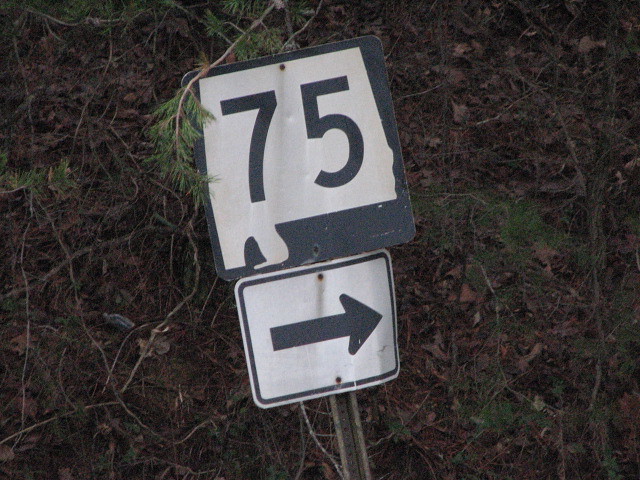In this outdoor photograph, the majority of the background features a wooded area with dense shrubbery comprised of branches, twigs, and patches of dark green grass. The ground is strewn with dry, brown leaves and broken branches. Prominently, at the center of the image stands a rusted metal post to which two street signs are attached. The upper sign is a white square with a black border, displaying the numbers "75" in bold black font. Beneath this, there is a smaller rectangular sign with a solid black arrow pointing to the right. The post appears to have been knocked over into the wooded area, leaning amidst the forested grass and dirt.